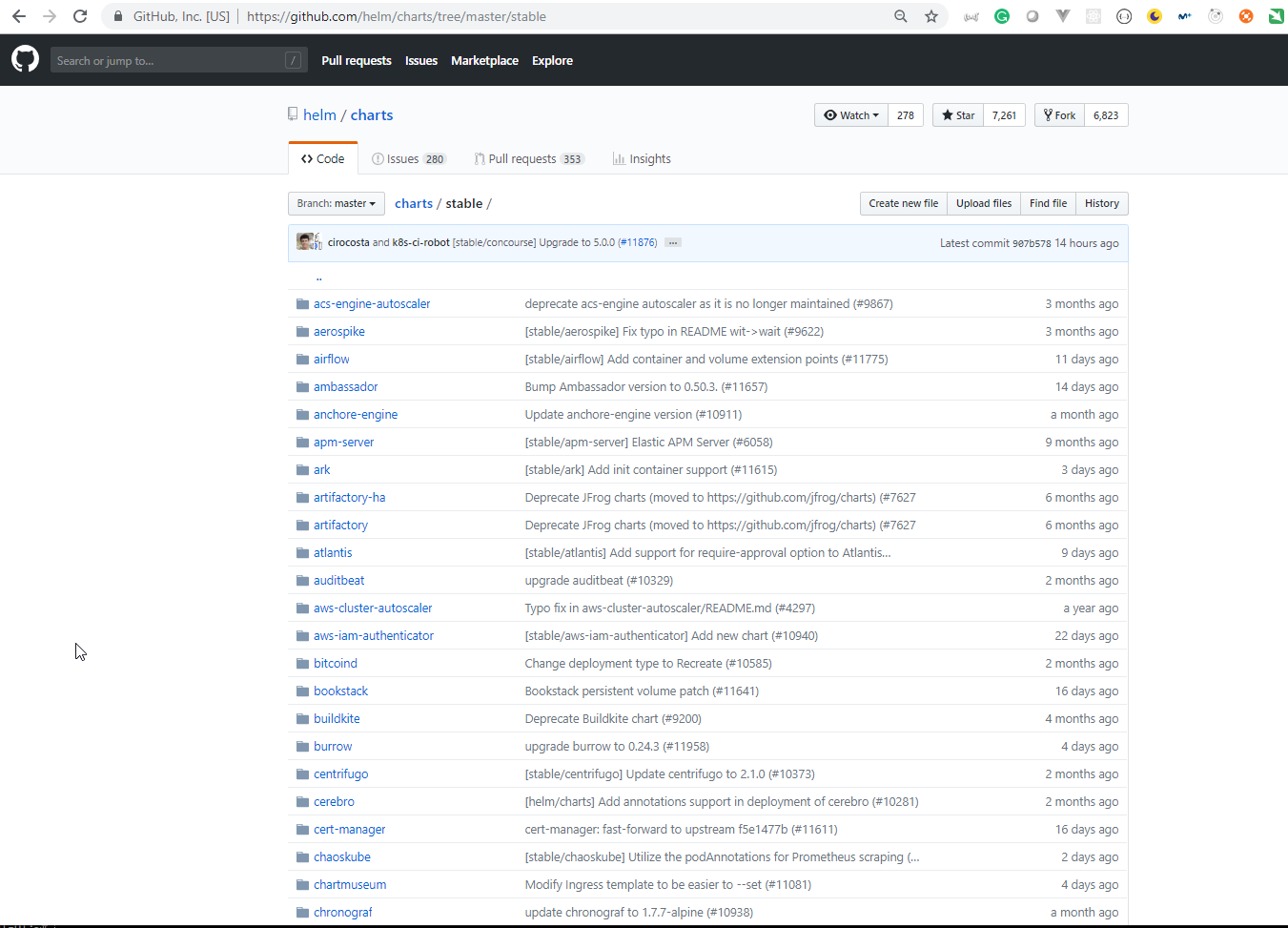In the image, the top portion features a gray background with the text "GitHub, Incorporated (US)" prominently displayed. Below this, a long black search bar is flanked by navigational options: "Pull requests," "Issues," "Marketplace," and "Explore." Below the search bar, there is blue text that reads "helm-charts."

Next, several tabs are available: "Code," "Issues," "Pull requests," and "Insights." Directly underneath these options are "Charts" and "Stable."

To the right, additional subcategories are presented: "Create new file," "Upload files," "Find me," and "History." Below these, approximately 20 clickable subcategories are listed in small, lowercase blue text with corresponding checkboxes beside them. Notable names among these subcategories include "arc," "burrow," and "court manager."

Farther to the right, links to issues or other content are visible, each accompanied by a timestamp indicating their age, ranging from "three months ago" to "one month ago."